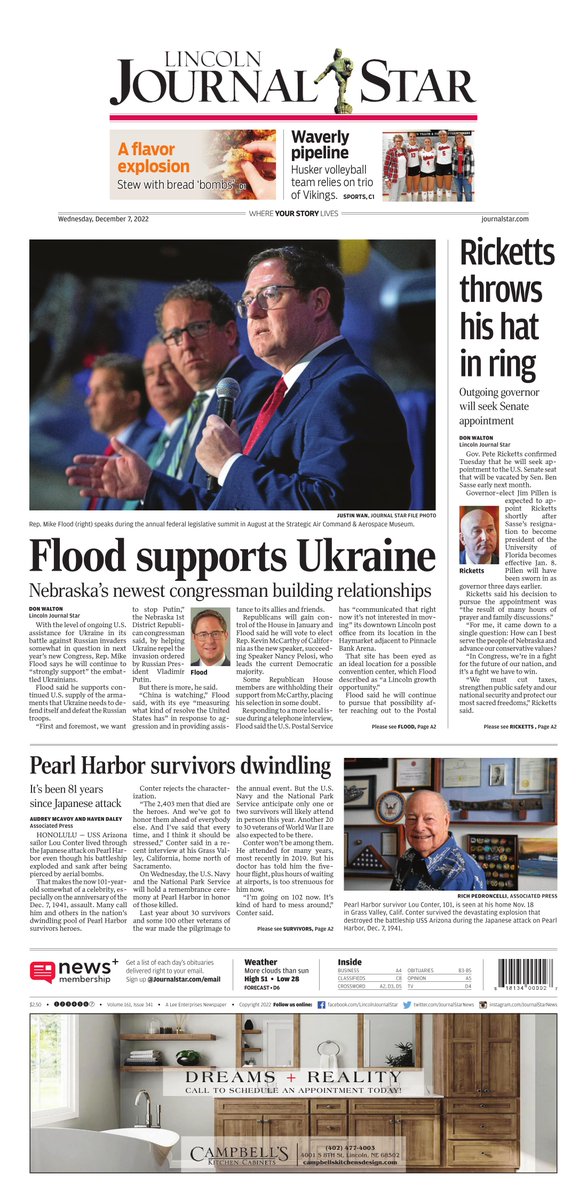This image captures the front page of the "Lincoln Journal Star" newspaper. At the top in bold black text, it reads "Lincoln Journal Star" with an icon of a pitcher getting ready to throw a ball situated between "Journal" and "Star." 

Beneath the header, there are two prominent images. The first, labeled in orange text as "A Flavor Explosion," showcases a person holding a piece of food. The second, under the black text headline "Waverly Pipeline," features an image of approximately five individuals.

Further down, the headline "Flood Supports Ukraine" appears, reporting on Nebraska's newest congressman's relationship-building efforts. Accompanying this headline is an image of four men in suits, two of whom are wearing glasses. 

Another notable headline reads "Ricketts throws his hat in the ring," alongside a photograph of a man with a bald head. This section includes two to three paragraphs of text.

Continuing down, there's a headline "Pearl Harbor Survivors Dwindling," complemented by about three paragraphs of text and an image of an elderly man. The elderly man, dressed in a blue shirt, is smiling with framed photos in the background.

Additional details include small blurbs in black text, a black barcode, and at the bottom, social media links for Facebook and Twitter. An inset image showcases a bathroom featuring light-toned cabinets, white walls, a white bathtub with a silver faucet, and a white window. This image is associated with the caption "Dreams, Reality."